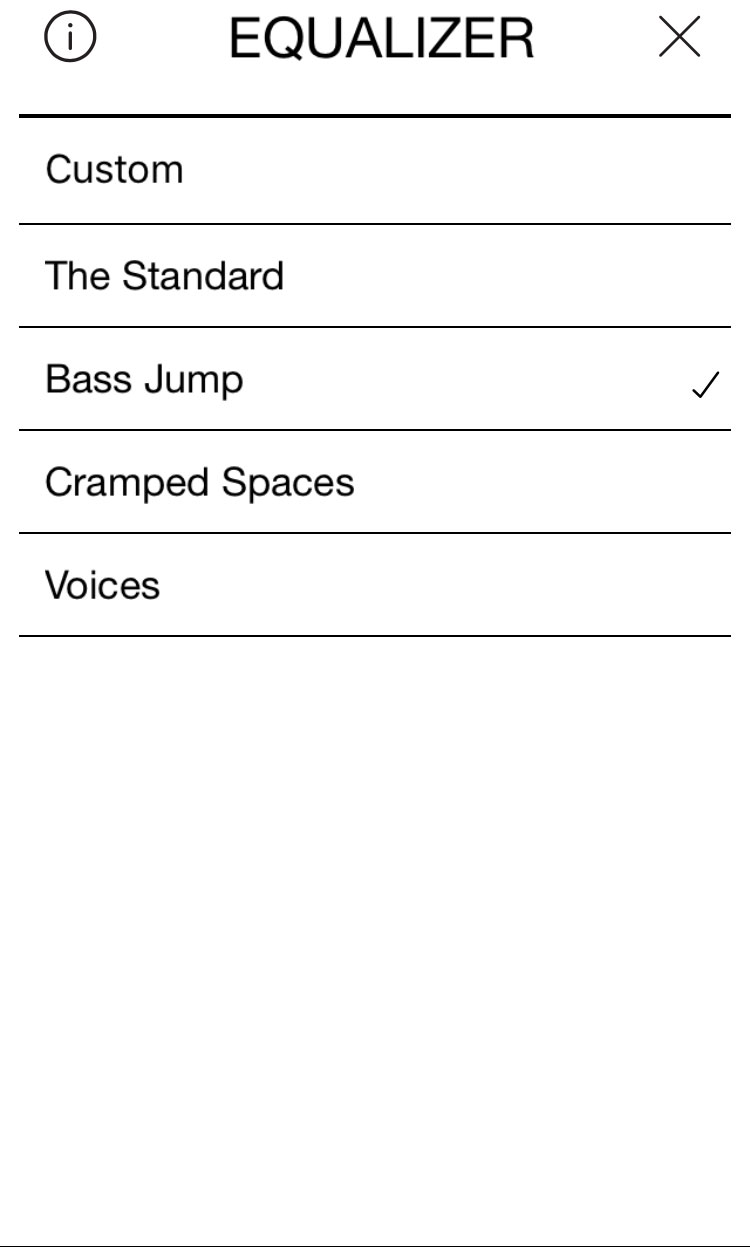The interface screen displays on a white background in portrait orientation. At the very bottom of the screen, there is a faint black horizontal line extending from left to right. In the top left corner, a circle with the letter "I" inside is present. Situated at the top center, the word "EQUALIZER" is prominently displayed in all capital black letters. On the top right corner, there is an "X" icon designed for closing the screen.

Directly beneath this header is a small space followed by a thick, bold black line stretching horizontally. Below this line, the word "CUSTOM" appears, with a proportional space separating the two. Another small space is present underneath "CUSTOM," followed by a thin, faint horizontal line. After a bit of vertical space, the word "STANDARD" appears. 

Continuing downward, more space precedes another faint horizontal line, followed by additional space. The term "BASS JUMP" is shown next, marked with a right tick (√) signifying its selection. Further down, another thin line is followed by a small space, leading to the phrase "CRAMPED SPACES." A little more space is followed by another thin line across the screen. 

After more space, the option "VOICES" is displayed. Beneath "VOICES," yet another thin black line extends from left to right. The lower portion of the screen is largely empty, only interrupted at the very bottom by another faint horizontal line.

The format suggests the interface is an equalizer settings menu, possibly part of music production software or an audio settings page on a digital device. The user evidently opted for the "BASS JUMP" setting.